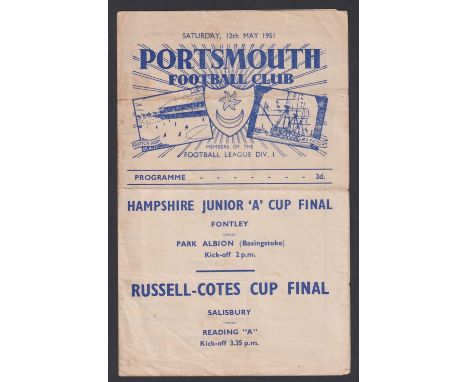This photograph features the cover of a Portsmouth Football Club program for the Hampshire Junior A Cup Final and the Russell-Coats Cup Final, dated Saturday, 12th May, 1951. The vertically rectangular program, outlined with a black frame and set against a light gray background, prominently displays "PORTSMOUTH" in large blue letters at the top, followed by "FOOTBALL CLUB" in slightly smaller blue text. Below this, there are three images: a drawing of a soccer field to the left, a central shield with a star and crescent moon, and an image of a ship to the right.

Under these images, the text "FOOTBALL LEAGUE DIVISION ONE" appears above a horizontal blue line. Below this line, the word "PROGRAMME" is printed to the left, followed by a series of dots, and "24" to the right. Another blue horizontal line separates this section from the next. The title "HAMPSHIRE JUNIOR 'A' CUP FINAL" follows, with "FONTLEY vs. PARK ALBION" beneath it and a kickoff time of 2.35 p.m. Divided by another blue line, the second title "RUSSELL-COATS CUP FINAL" is displayed, with "SALISBURY vs. READING 'A'" below it, concluding with a kickoff time of 3.35 p.m.